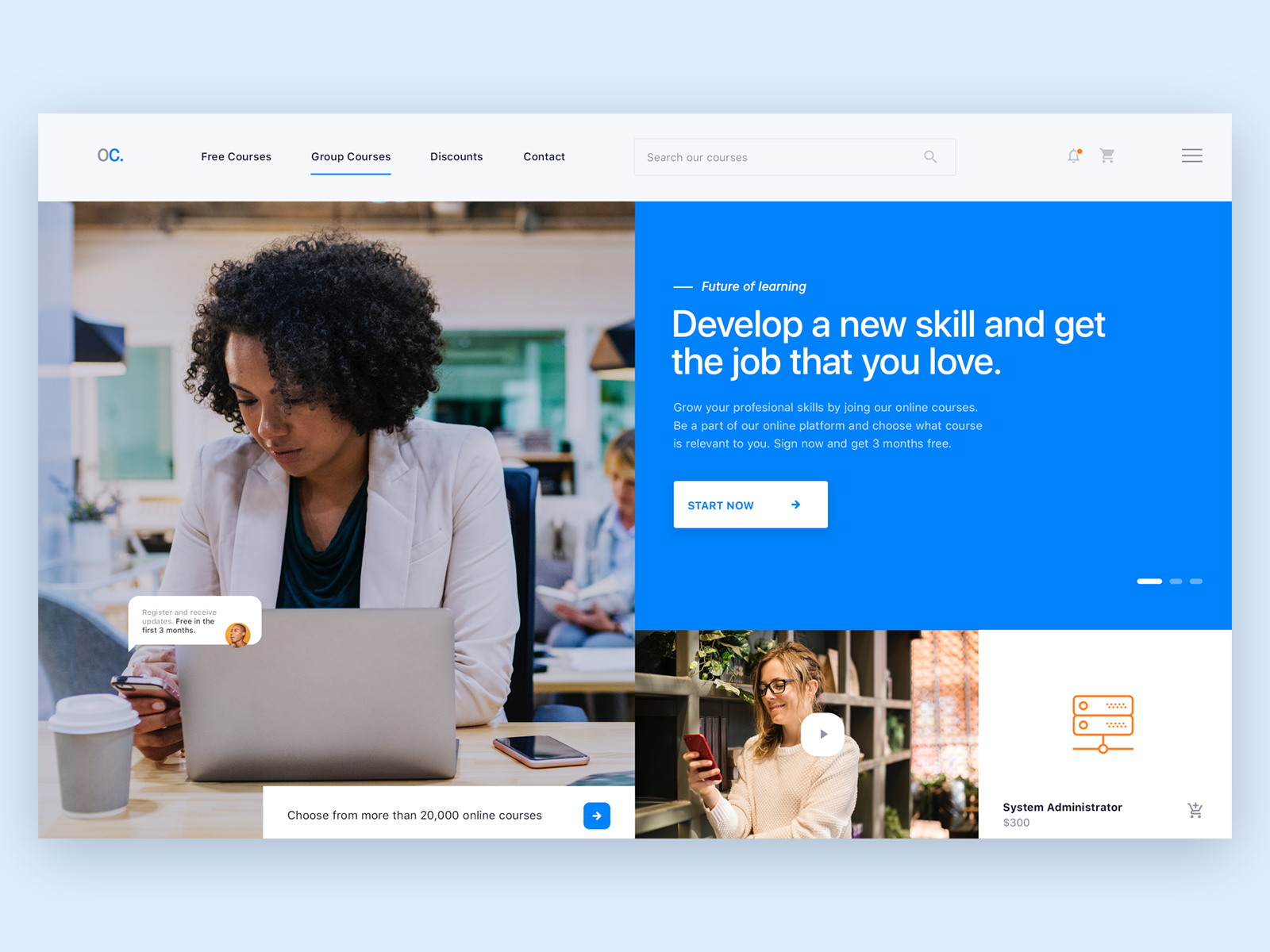**Image Description:**

The background of the image is a light blue color. Superimposed on this background is a white rectangle located towards the left-hand side of the image. Inside this rectangle, there is a large gray "O" next to a blue "C," both followed by a small blue period. Below this, the words "Group Courses" are displayed in black, with capital letters for the initial of each word. The words are underlined in blue. 

Beneath this text is the label "Discount and Contact." A white search box outlined in gray is present on the right side, containing the text "Search All Courses" in gray with a capital "S." Adjacent to this search box are icons, including a gray bell with an orange notification circle, a gray shopping cart, and three stacked gray lines representing a menu.

Below these icons, there's an image of a woman with black curly hair, wearing a white blazer over a teal-colored shirt, holding her phone. A text box near her phone displays the message: "Register and receive updates and sales free for the first three months" in gray text on a white background.

The woman is also using a silver laptop. Below the laptop, there is black text that reads: "Choose from more than 20,000 online courses" with a white arrow pointing to the right. 

In addition to this, there is a gray label stating "$300" near the phrase "Future of Learning." The image includes the text: "Develop a new skill and get the job that you love. Grow your professional skills by joining our online platform and choose what course is relevant to you. Sign up now and get three months free." It should be noted that the word "joining" is misspelled as "joing."

Overall, the image promotes an online learning platform, emphasizing the availability of extensive courses and special offers for new users.